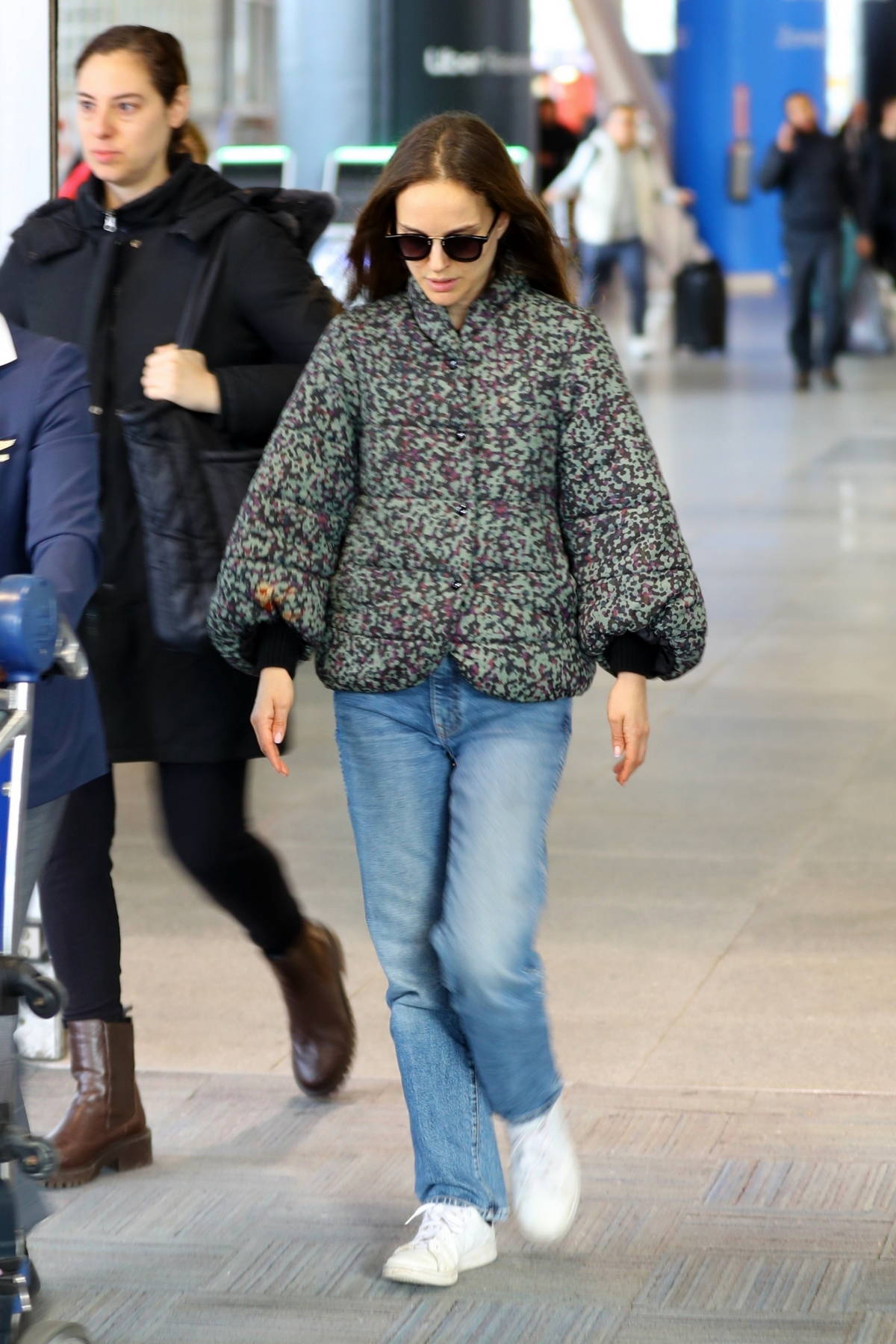In the center of this image, a young woman stands as the focal point, seemingly captured in an airport setting. She wears a distinctive puffy jacket featuring a green and purple print, paired with blue denim jeans and white sneakers. Her long brown hair flows behind her back as she looks downward, her face partially obscured by large black sunglasses. Walking close behind her, another woman is dressed entirely in black, including a black coat, pants, and shirt, complemented by brown Chelsea boots and carrying a black handbag. The scene takes place on a light brown tiled floor, with a blurred background bustling with travelers and various colors such as black, white, gray, silver, and shades of blue, purple, green, red, and pink. Despite some text visible in the blurred background, it remains indecipherable. The image captures a moment of movement and anonymity, characteristic of busy airport terminals.